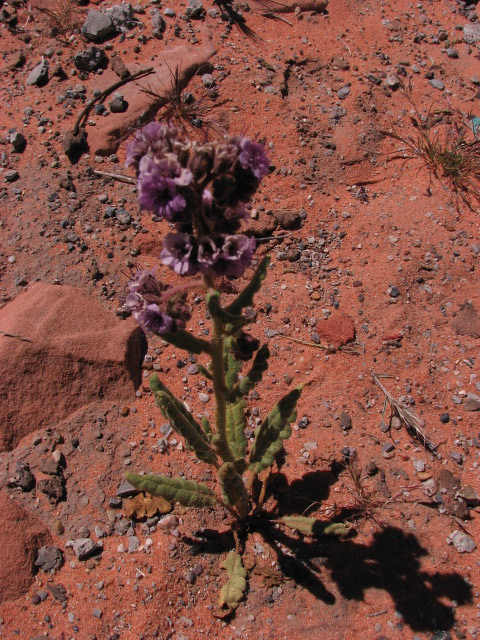This photograph captures a vibrant scene of a green cactus plant adorned with delicate purple flowers, which are lavender and white in color, blossoming at the top. The setting is an arid desert landscape, bathed in daylight, with the plant casting a distinct shadow on the reddish-brown, sandy soil. Scattered across the ground are numerous pebbles and rocks, varying in shades of gray and brown and presenting a sharp, jagged appearance. The dry soil is interspersed with scraggly bits of grass, particularly noticeable in the top right corner of the image, where more rocks are visible behind the grass. Additionally, a black and gray feather lies on the bottom right side, near the cactus, adding a unique element to the rugged terrain. The overall scene exudes a harsh yet striking beauty, emphasizing the contrast between the sharp, dry environment and the soft, delicate blooms of the cactus.